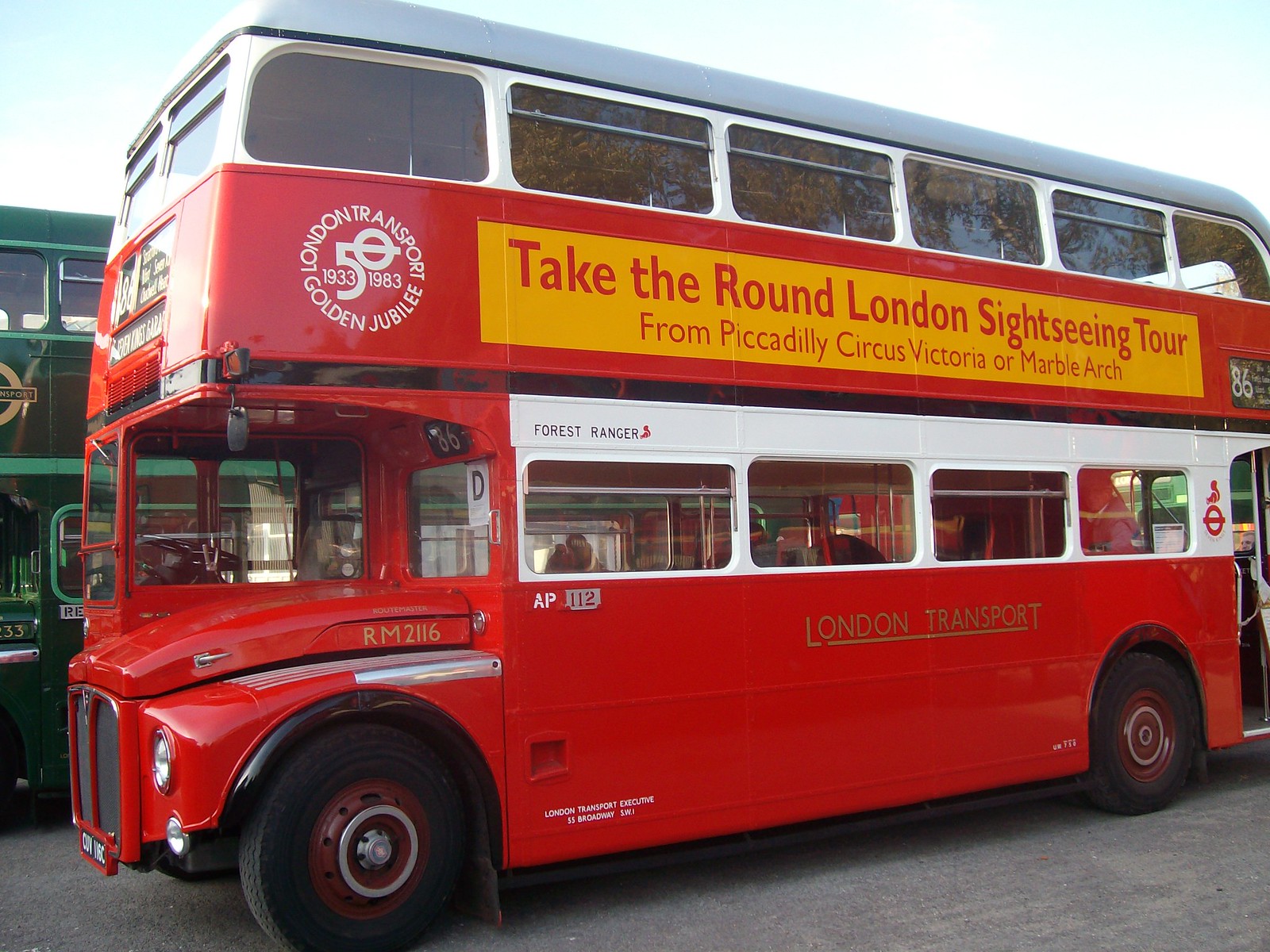This full-color outdoor photograph, taken on a sunny day, features a classic red double-decker bus, facing left, with vibrant details that evoke a strong sense of nostalgia. The driver’s enclosed compartment is on the right side in front of the bus. This beautifully preserved vehicle bears the hallmark designs of the London Transport system, with the lower portion of the bus painted a bold red, and windows outlined in white. 

Prominently displayed on the side, a gold logo marks the "London Transport 50th Golden Jubilee," celebrating the years from 1933 to 1983, accompanied by the fleet number RM2116. Spanning across the side of the bus, a large yellow banner with red text invites onlookers to "Take the Round London Sightseeing Tour from Piccadilly Circus, Victoria, or Marble Arch." The upper deck features a white section beneath its roof, while the roof itself is grey. In the distance, a less visible green bus lurks, giving a nod to the diversity of the London fleet. The image’s bright blue sky overhead adds to the charm of this historic moment preserved in time.